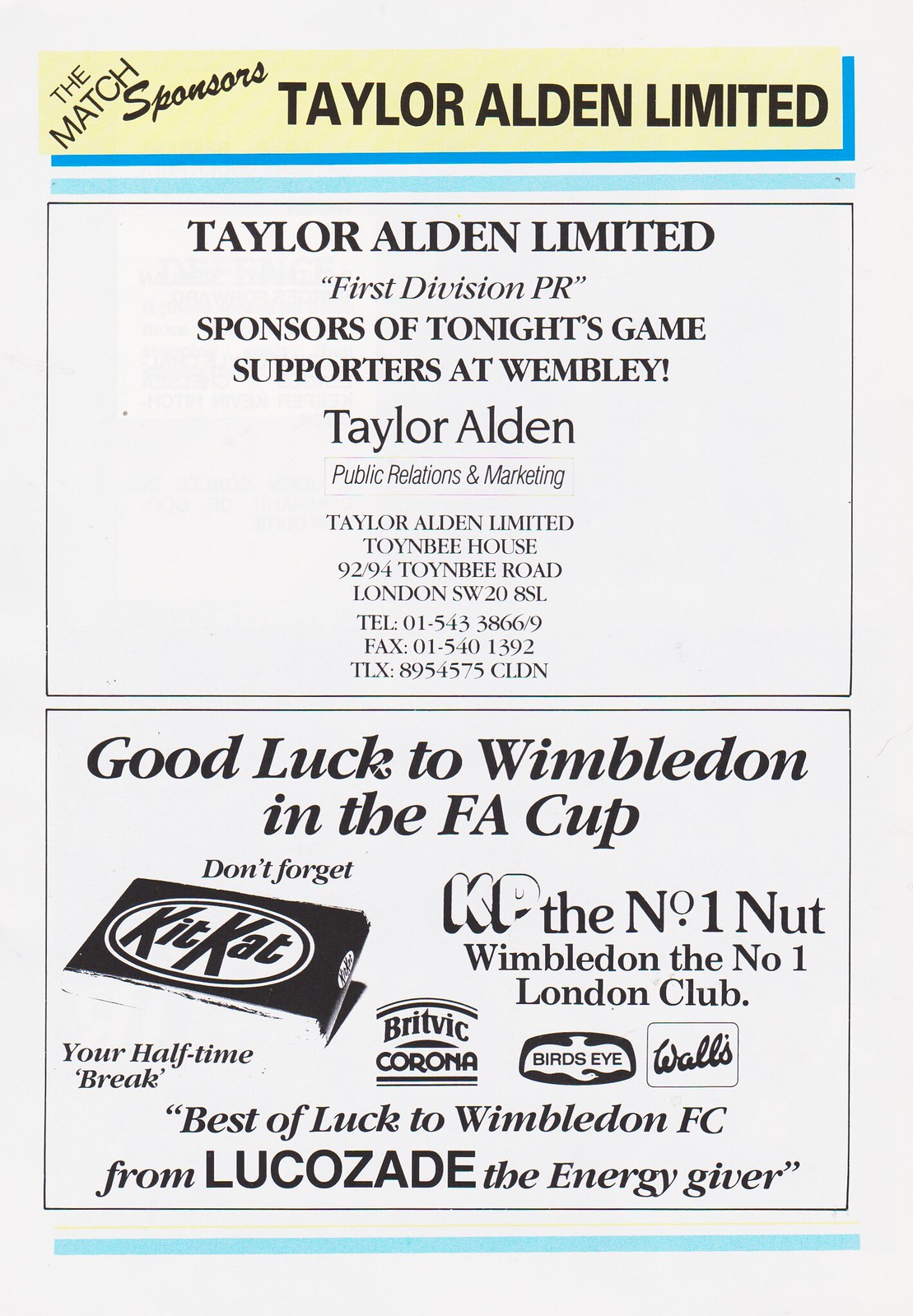This photograph captures a detailed page from a program featuring two rectangular advertisements stacked one above the other. The top advertisement prominently highlights the match sponsors, Taylor Alden Limited, showcasing their association as First Division PR sponsors of the game and supporters at Wembley. The ad lists their full address, Taylor Alden Limited, Toynbee House, 9294 Toynbee Road, London, SW 20SSL, along with their telephone number 01-513-38669. 

The bottom advertisement is a compilation of good luck messages to Wimbledon FC, wishing them success in the FA Cup. It features a variety of brands including Kit Kat, encouraging it as the ideal halftime break, KP, celebrated as the number one nut, and hails Wimbledon as the premier London club. Additional best wishes are extended from brands such as Britvic Corona, Birdseye, Walls, and Lucozade, termed the energy giver.